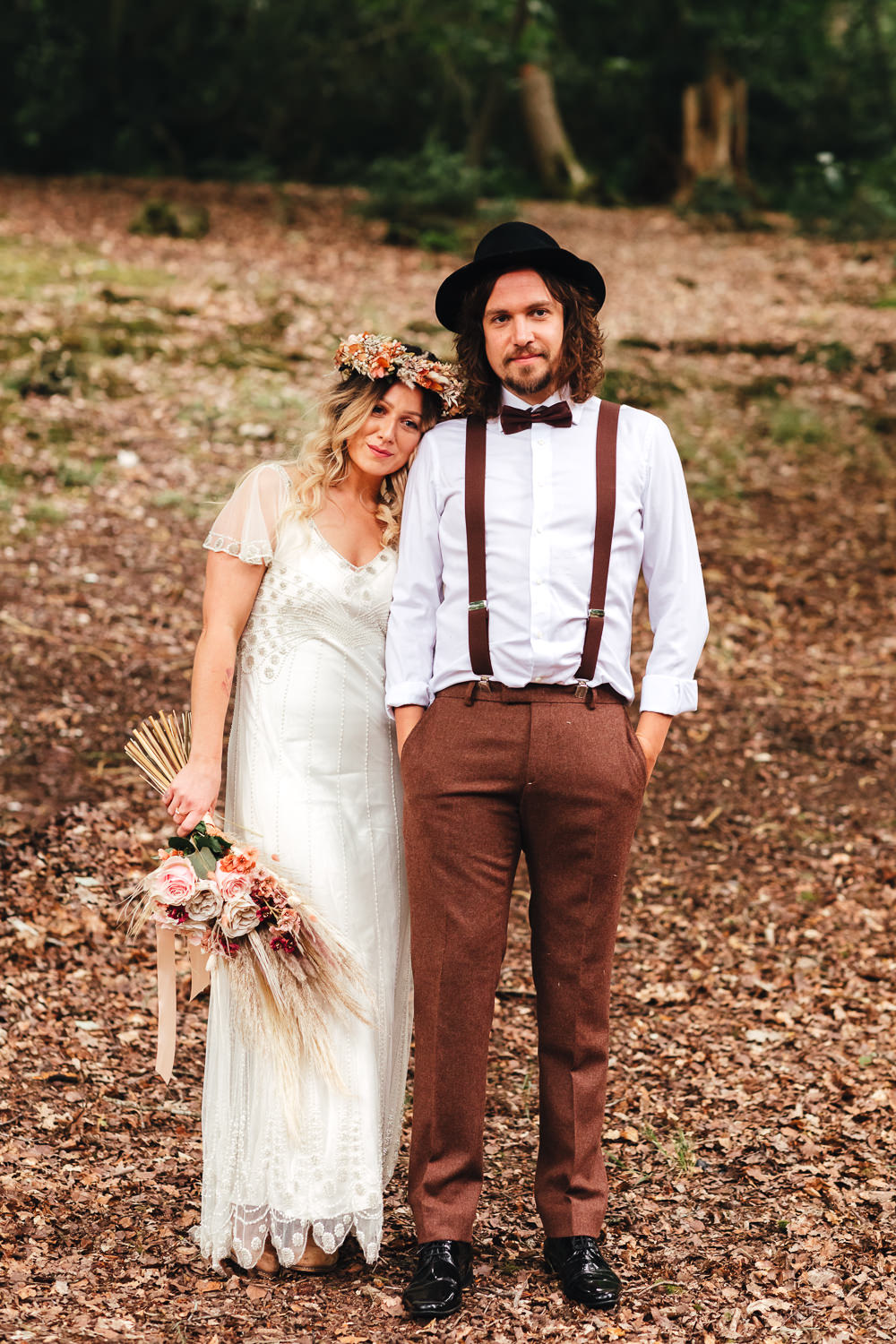In this outdoor color photograph, captured in portrait mode, we see a bride and groom standing amidst a ground strewn with brown leaves. The soft-focus background reveals dark green trees, creating an enchanting woodland setting. Positioned on the right, the groom is dressed in brown pants paired with matching suspenders and a white long-sleeved shirt. He adds a touch of elegance with a dark bow tie and a dark brimmed hat, while his curly shoulder-length hair frames his closely cropped mustache and beard. His shiny black shoes complete the ensemble, and he gazes directly at the camera with a composed expression.

On the left, the bride looks ethereal in an ivory-colored, cap-sleeve, long dress adorned with a scalloped hem. Her wavy blonde hair cascades past her shoulders, crowned with a delicate wreath of flowers and baby's breath. She cradles a bouquet composed of pinkish-brown roses, intertwined with cream-colored elements resembling wheat, all tied together with light brown ribbons that cascade downward. The bride leans affectionately against the groom's shoulder, adding a touch of intimacy and tenderness to the scene. This idyllic moment encapsulates the couple's rustic and romantic allure.